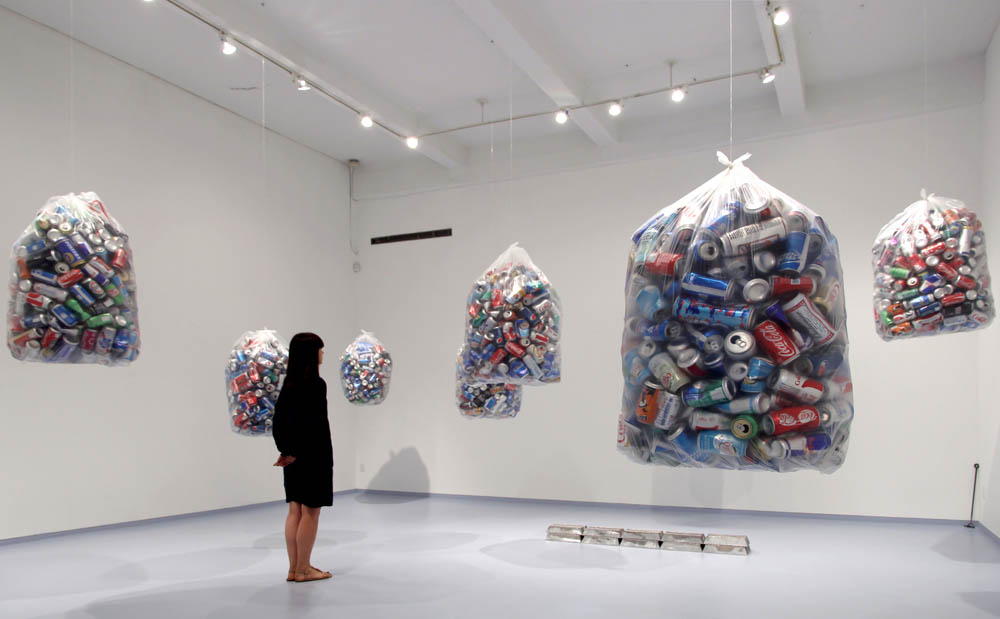In this detailed depiction of an art exhibit, a woman with dark hair, barefoot and dressed in a black dress, stands in a pristine white room. Her back is turned toward the viewer, focusing on the exhibit in front of her. The room, which appears to be an art gallery, is characterized by its white walls, white floor, and track lighting attached to metal beams on the ceiling. Hanging from the ceiling by white strings are seven transparent trash bags filled with a varied assortment of aluminum cans, including recognizable brands like Coca-Cola and possibly Budweiser, alongside other blue, white, and red cans. On the floor lie ten objects resembling silver and brownish bricks, stacked in a formation that suggests gold bars, though their exact material is unclear. In the right-hand corner of the room stands a tall, skinny black object, adding another layer of intrigue to the minimalist yet thought-provoking installation.